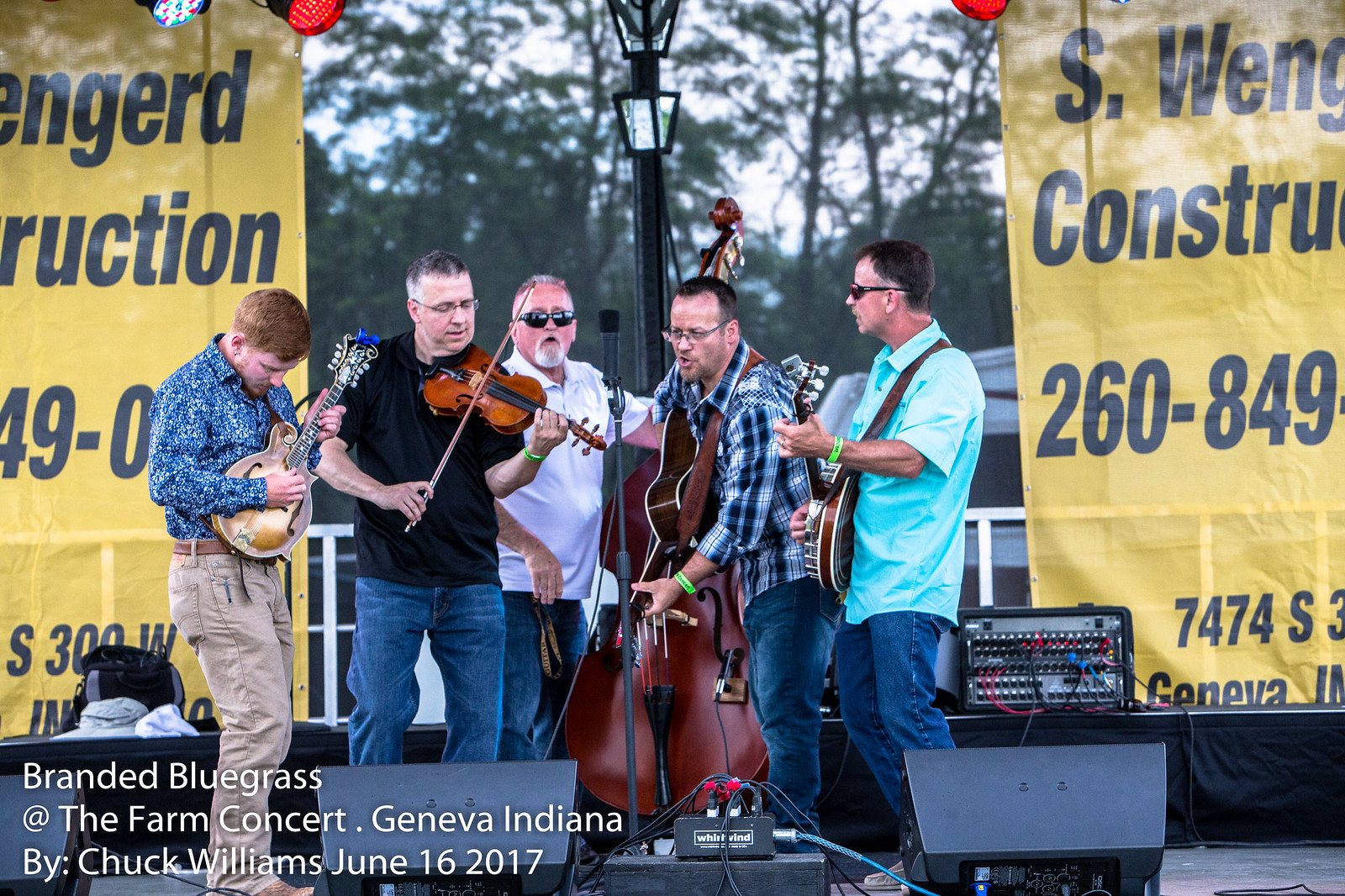This image, taken during the daytime, features an outdoor musical performance set against a backdrop of trees that suggest a forested area. The sky is visible above, with a lamp post subtly marking the location. Centrally framed is an open-air stage adorned with two yellow banners featuring some black writing, but the details are partially obscured. These banners flank the stage, one on the left and one on the right, and above them hang multicolored disco lights, suggesting a lively event.

On the stage are five male performers, each playing distinct instruments. From left to right: the first musician, dressed in a blue shirt and light brown trousers, with brown hair, holds what appears to be a golden small guitar or mandolin. Next to him is a violinist wearing blue jeans and a black t-shirt. The central figure, a white man with a white French beard and sunglasses, wears a white t-shirt and blue jeans while playing a large cello. To his right stands a vocalist and bass guitarist, bespectacled and clad in a blue and white shirt with blue jeans. The performer on the far right, also wearing sunglasses, dons a sky blue shirt and blue jeans as he strums a guitar.

All musicians wear green wristbands, suggesting perhaps event access or group identification. Equipment and wires are arranged on the stage, converging at the bottom right, and a microphone stands at the center of the group. The bottom left corner of the image features text in white lettering: "Branded Bluegrass at the Farm Concert, Geneva, Indiana by Chuck Williams, June 16, 2017." This caption provides key details about the event and its documentation.